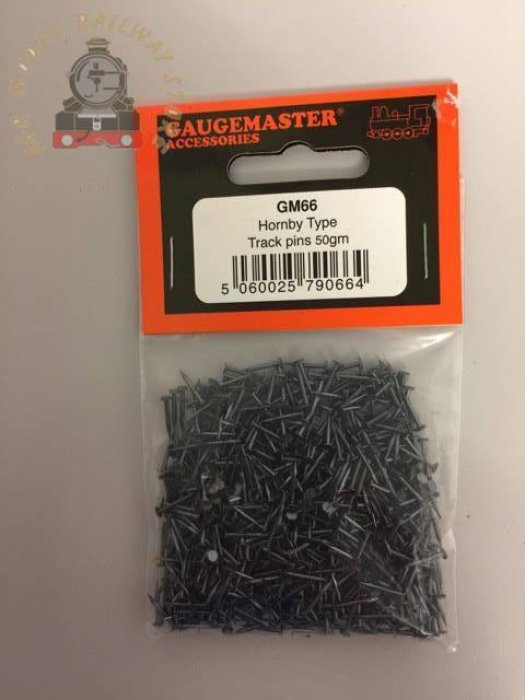The image showcases a clear plastic bag containing hundreds of small black track pins, approximately an inch long. These pins are used for securing miniature model train tracks. The bag prominently features an orange and black stapled label, with the top displaying "Gage Master Accessories" in orange text. Adjacent to this text is an intricate illustration of an old steam train from the 1800s. The label also includes the description "GM 66 Hornby type, Track Pins 50 GM" inside a white boxed section, along with a barcode (5060025790664) near the bottom. The background of the image appears pinkish-tan, though it might be slightly dark. Additionally, there's a faint watermark reading "Railway Store" accompanied by a ghostly train image, adding a unique touch to the overall appearance.